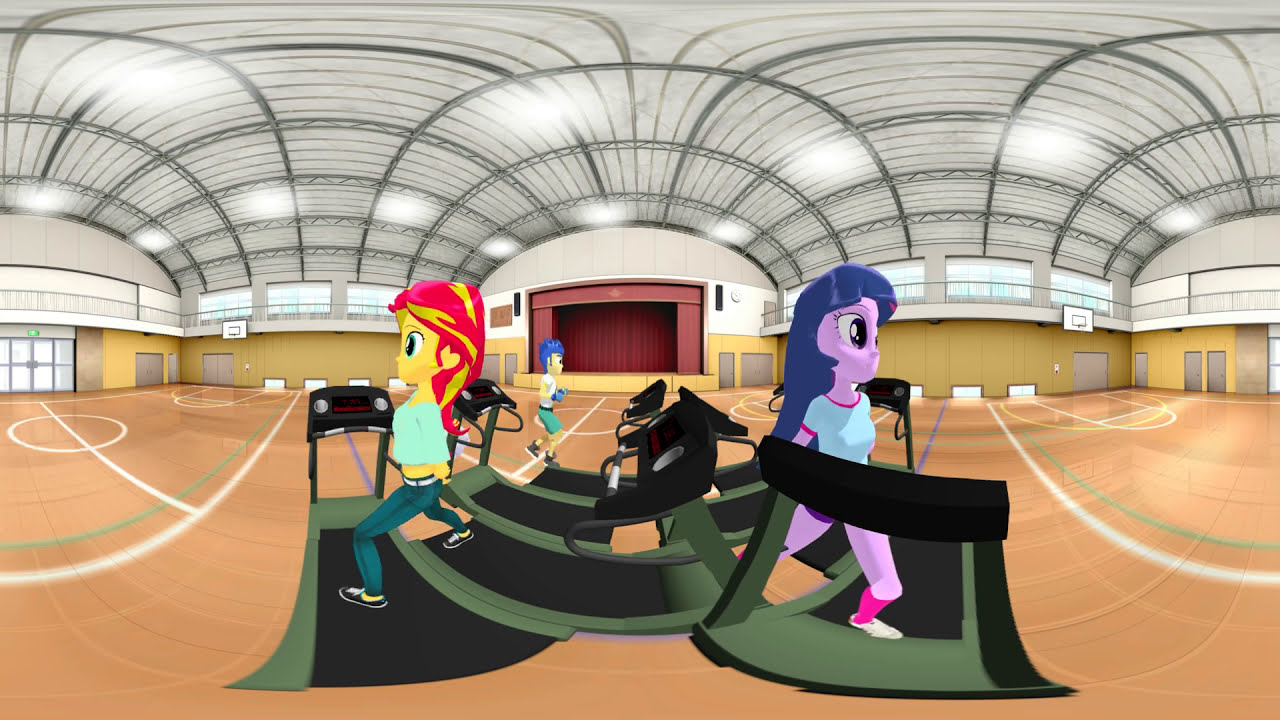The image depicts a peculiar cartoon scene set in a gymnasium with a basketball court, captured in a fisheye lens effect. At the center of the court, two My Little Pony characters, seemingly anthropomorphized into women, are exercising on overlapping treadmills. The character on the left has purple skin, bluish-purple hair, a green shirt, pink pants, and pink socks. The character on the right has yellow skin, red and yellow hair, a green shirt, and green pants. A third character, who does not resemble the My Little Pony characters, is seen walking around. The gymnasium features a metal-framed ceiling with lights, curved arches, and walls painted yellow, adorned with glass and metal doors. The court markings are distinct, with a central circle and key areas clearly outlined. There is also a red stage with a curtain visible in the background. The floor is a light brown color, and no one is engaging in basketball, as exercising seems to be the main focus of this animated scene.